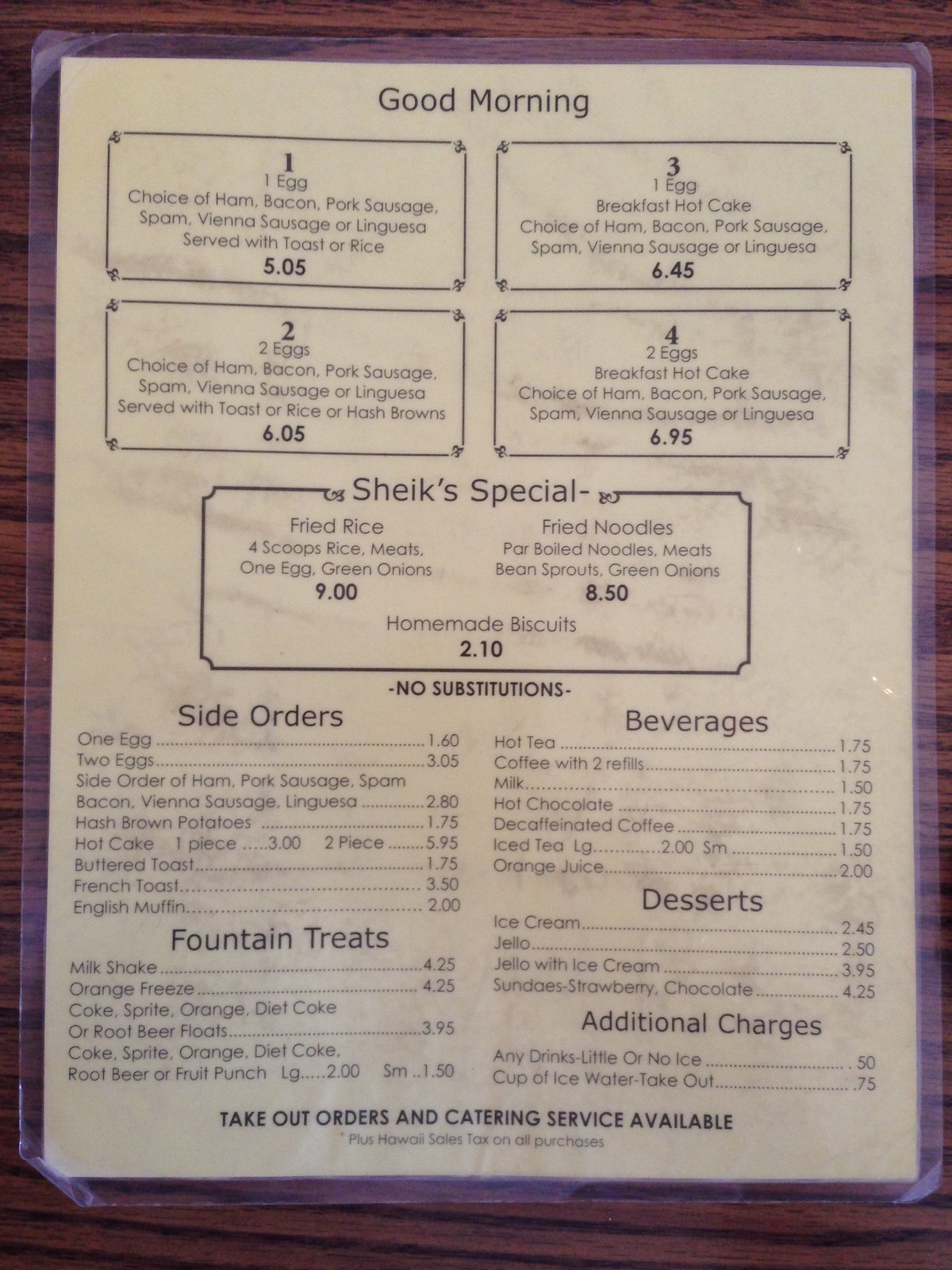This image captures a white laminated menu displayed prominently on a dark brown, horizontal woodgrain table. The menu's header, "Good Morning," is featured in bold black letters at the top center. Beneath this greeting are four distinct breakfast dishes listed, each encapsulated in a long rectangular box with detailed descriptions and pricing.

- **Item 1:** Positioned directly under "Good Morning" on the top left, this box includes a single egg with accompanying sides. Its price, $5.05, is printed at the bottom of the rectangle.
- **Item 2:** Found beneath Item 1, this box lists the items included in the second dish, with the price set at $6.05.
- **Item 3:** To the right of Item 1, this box details the third breakfast option, costing $6.45.
- **Item 4:** Located below Item 3, this box lists the components of the fourth dish alongside its price.

Centrally aligned below the boxes for Items 2 and 4 sits "Sheik's Special," flanked by additional breakfast items:
- **Left Side:** Fried rice, with its respective price.
- **Right Side:** Fried noodles, also paired with a price.

Beneath both of these, the words "homemade biscuits" appear, followed by the cautionary note, "No Substitutions," in small black letters. The lower half of the menu is divided into two sections:

**Left Section:**
- **Side Orders:** Contains approximately 10 items with their prices listed to the right.
- **Fountain Treats:** Lists around 7 items beneath.

**Right Section:**
- **Beverages:** Includes about 7 drink options, each priced accordingly.
- **Desserts:** Features 4 dessert options in bold black letters.
- **Additional Charges:** Outlines two specific items under this heading.

Spanning the bottom of the menu in large black lettering is the notice: "Takeout Orders and Catering Services Available."